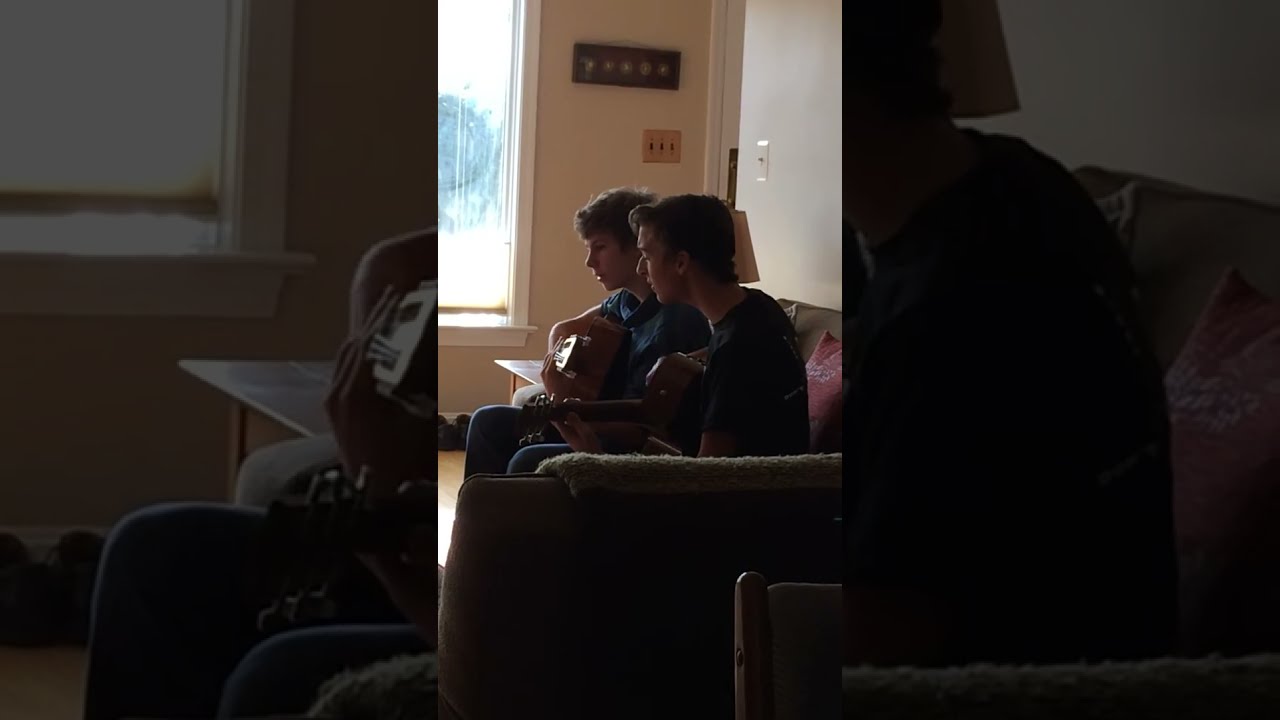In a cozy living room setting, a photograph captures two young men seated side by side on a brown loveseat with a red cushion at the back. Both are engrossed in playing acoustic guitars. The man on the left, who appears to be in his late teens, has short, curly brown hair and wears a short-sleeved black t-shirt. He is singing, his face partially hidden as he looks down at his guitar. Next to him is a slightly younger-looking man with short hair, who dons blue jeans and a green and blue striped collared shirt. He, too, is focused on his guitar, looking downward. The scene is gently backlit by sunlight streaming through a window behind them, casting a soft glow against the off-white wall, which features an electrical outlet. The hardwood floor adds a warm, light brown hue to the setting, enhancing the intimate, daytime atmosphere of the living space.